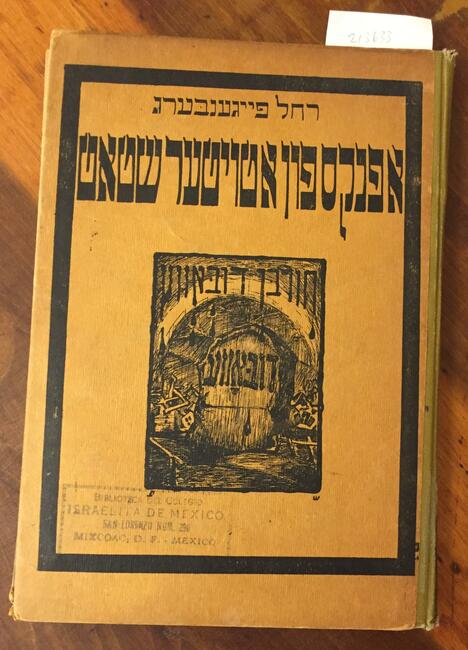This image depicts an old, worn book lying flat on a wooden table with a yellowish hue. The book's cover is light tan and features black inscriptions in an unfamiliar, possibly Semitic or Hebrew, language. The book's binding is visible on the right, suggesting it opens from right to left, characteristic of Hebrew texts. The cover includes an image of what appears to be a wooden gate, possibly in a cave system, though this detail is somewhat ambiguous. Additionally, there is a noticeable stamp on the cover that reads "Israelethetamehico," hinting at a potential connection to Mexico, perhaps indicating the book's current location rather than its origin. The overall state of the book, with its worn and aged appearance, adds a sense of historical significance to the artifact.